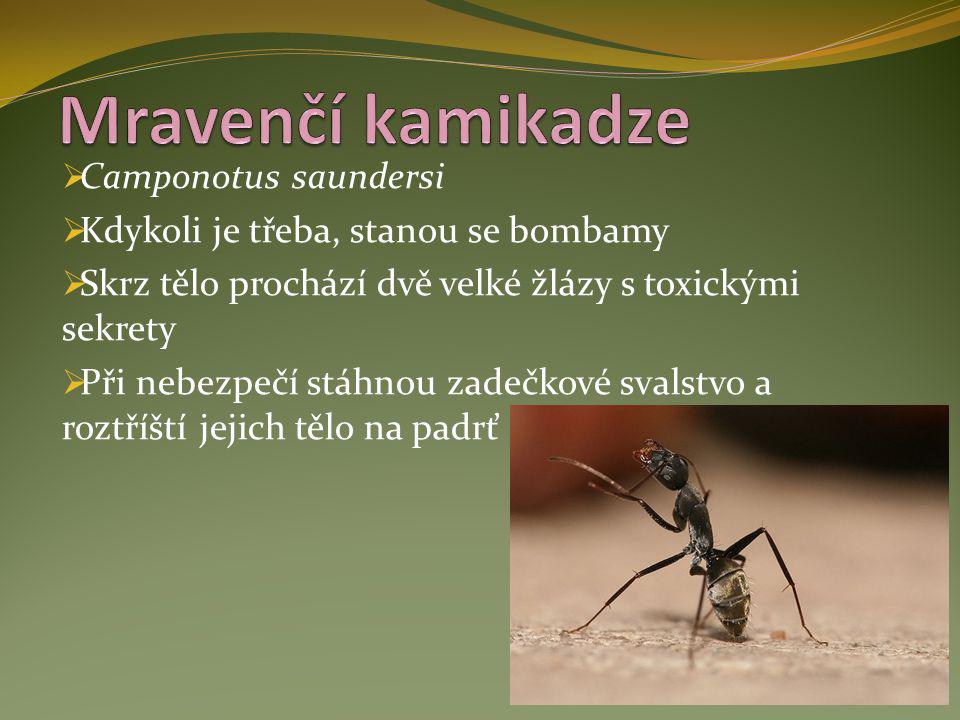The PowerPoint slide titled "Mravenci Kamikadze" features a light purple heading and four bullet points in white text, written in what appears to be a foreign language. The bullet points are as follows:

1. Camponotus Sondersi
2. Kadaikoli J. Treba, Steno se Bombay me
3. Skars Telo Prochazi Due Velke Zlezi S. Toxic Chimey Security
4. Prai Nebes Pesi Steno Zadek Kove Svalstvo E. Rostristi Jecic Telo Na Padart

The background of the slide is predominantly green with a wavy pattern in yellow and orange at the top. In the lower right corner, there is a close-up image of an ant standing on its back four legs, with its front legs and head raised, looking towards the top right. The ant is positioned on a tan surface, possibly a rock.